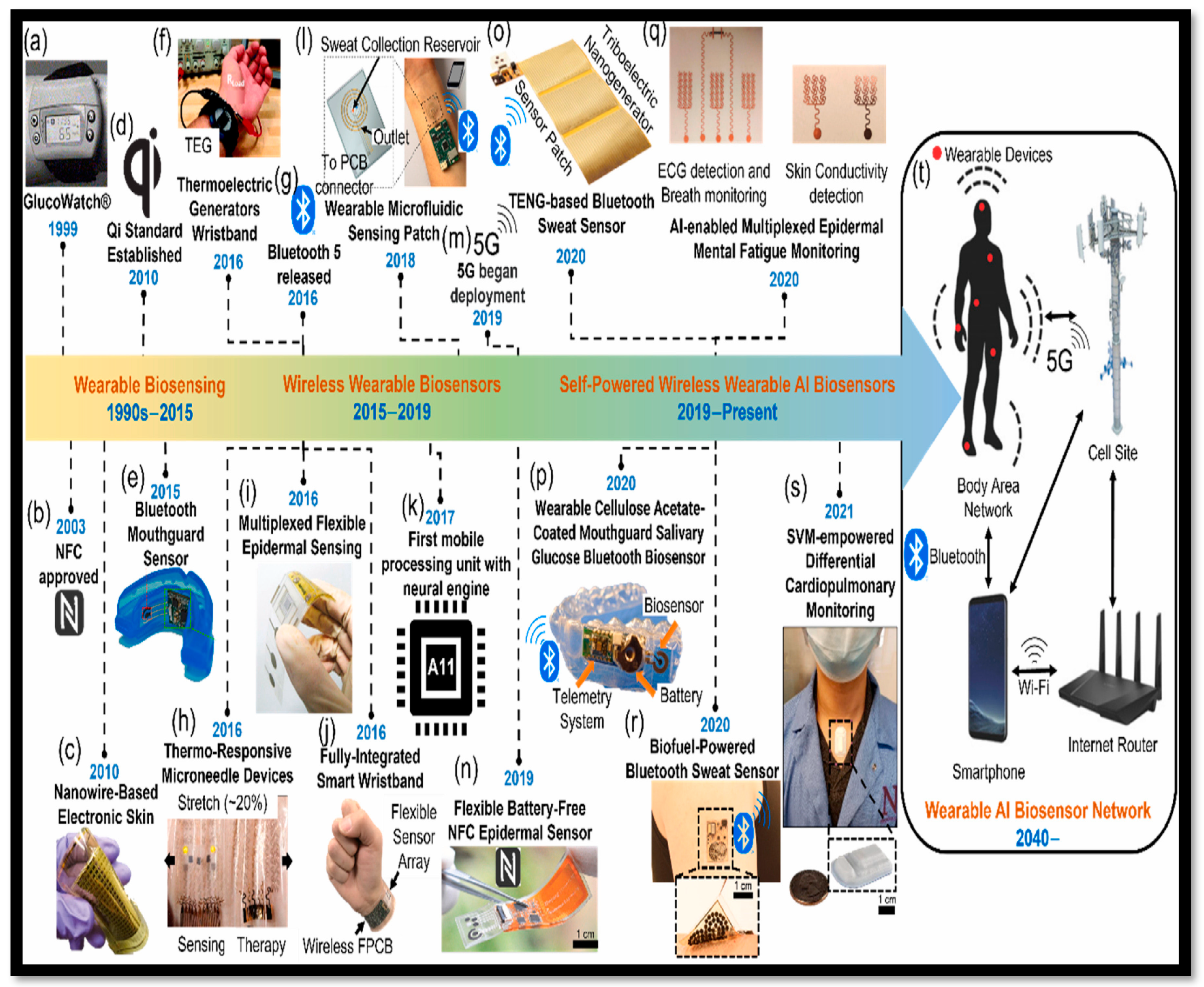The image is a detailed and colorful diagram depicting the progression of wearable biosensing technology from the 1990s to the present. The central feature is a horizontal arrow labeled with dates and technological milestones, dividing the timeline into three segments: "Wearable Biosensing (1990s to 2015)," "Wireless Wearable Biosensors (2015 to 2019)," and "Self-Powered Wireless Wearable AI Biosensors (2019 to Present)." Various small images and illustrations are positioned above and below the arrow, each representing different types of biosensing devices. These include NFC-approved devices like those used in Apple Pay, 5G cell towers, smartphones, and routers. 

The diagram also highlights several specific wearable gadgets such as a Video Wristband, Theromatic Generator Wristbands, Ting-Based Bluetooth Sweat Sensor, Wearable Microfluid Sensing Patch, Glucose Monitoring Watch, Thermal Responsive Microneedle Devices, Fully Integrated Smart Wristbands, Nano Wire-Based Electronic Skin, and a Mobile Processing Unit with Neural Engine. These devices feature sophisticated technologies like Bluetooth, Wi-Fi, conductivity detection, and thermal responsiveness, showcasing the innovation and advancement in wearable biosensing tech over the years.